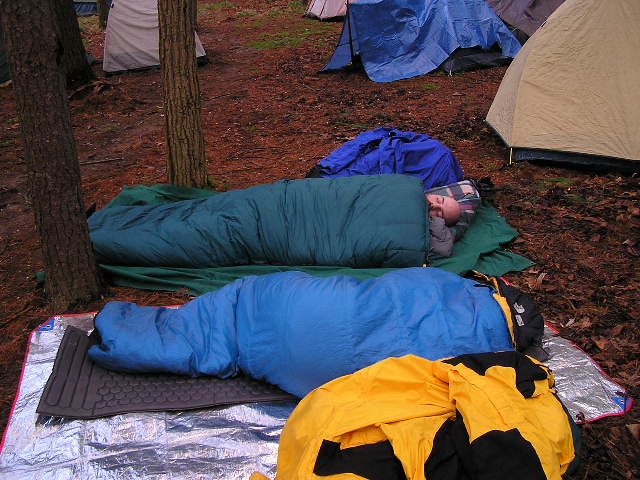The image depicts a bustling campsite set on a dirt ground sprinkled with a few brown leaves and encircled by towering tree trunks. In the foreground, a blue sleeping bag rests atop a reflective silver blanket and a gray mat, hinting at a cozy sleeping arrangement. Adjacent to this, a man lies facing the camera in a green sleeping bag on a green blanket. Additional sleeping bags, including a distinctive yellow and black one, are scattered across the terrain, suggesting more campers nestled in for the night. In the back right corner stands a pump tent, with a beige canvas tent and a small blue tent nearby. The camp area is dotted with various individual-sized tents, all set up on the plain dirt and wood-covered ground, enhancing the scene's rustic, outdoor ambiance.